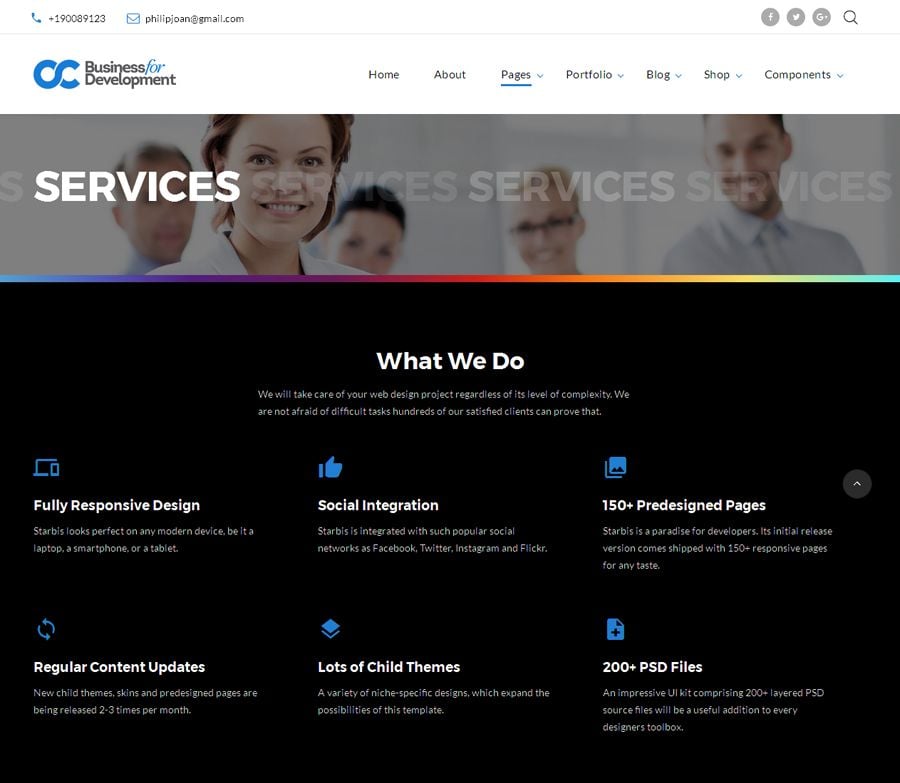A comprehensive screenshot of a business development service's website is presented, highlighting their extensive offerings and contact information. At the top of the page, the contact details are prominently displayed: a phone number (+1 900-89123) and an email address (philipjohn@gmail.com). The company’s logo, "Business for Development," featuring a stylized “BC” icon, is situated on the left.

The website’s navigation menu includes the following options: Home, About, Pages, Portfolio, Blog, Shop, Components, and a Search icon. Below the menu is a prominent main banner image showing smiling professionals. Overlaid on this image is the repeated word “Services” in large, semi-transparent text.

The central text in the banner states: "What do we do?" followed by details of their key offerings: "Fully responsive design," "Social integration," "150+ pre-designed pages," "Regular content updates," "Lots of child themes," and "200+ PSD files." These features showcase the company's expertise in web design, social media integration, regular updates, and providing a wide variety of pre-designed pages and child themes to meet client needs.

The image and text together effectively highlight the company's focus on delivering comprehensive development solutions, aiming to attract potential clients looking for thorough and modern business development services. The website’s name, "Business for Development," is repeated for emphasis.